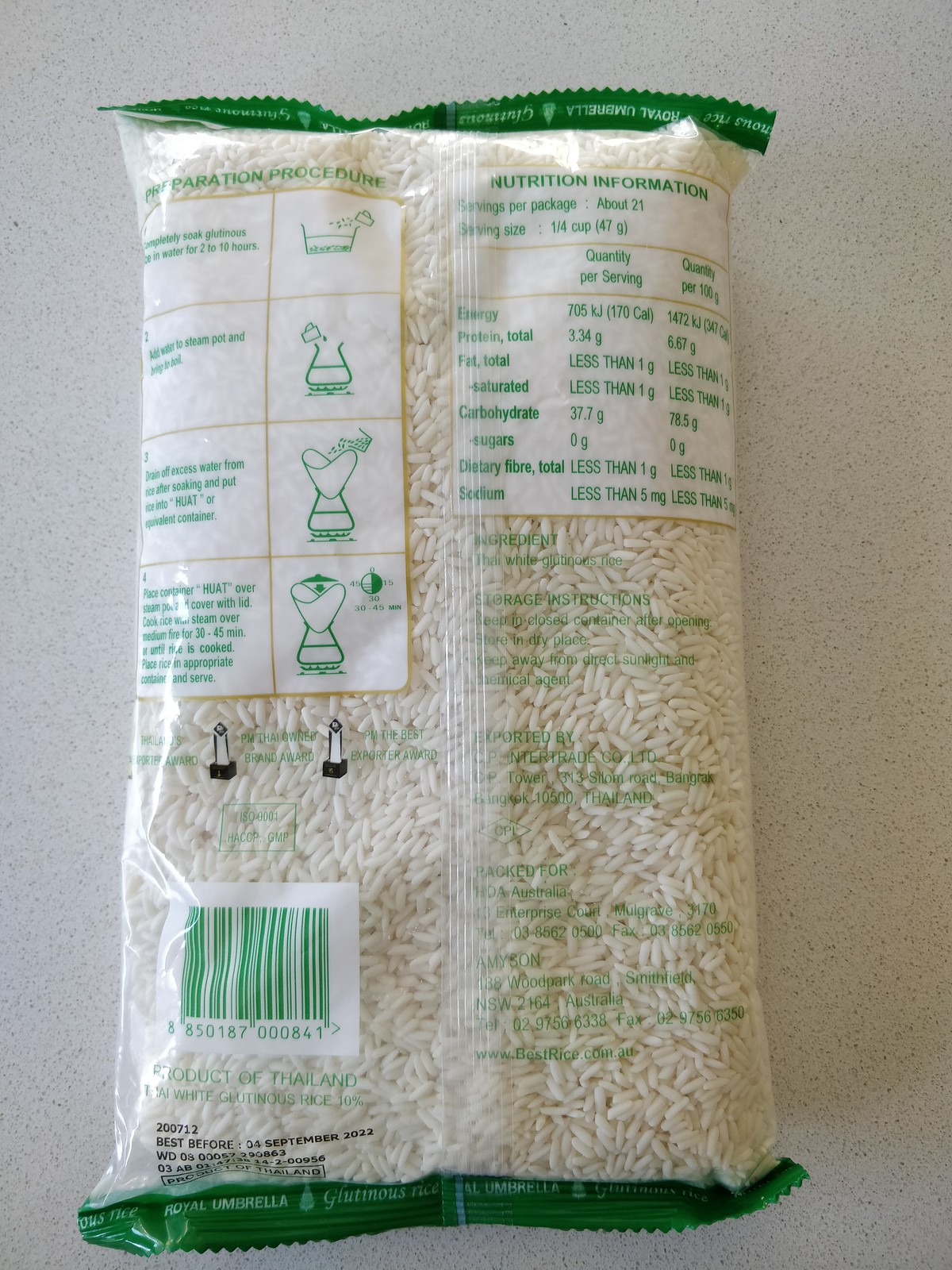This photograph features an inverted package of rice placed on a white granite countertop speckled with black accents. The image captures the back of the rice package, detailing the cooking instructions and nutritional facts. Specifically, the nutrition label reveals there are 21 servings per package, with each serving size being 47 grams (1/4 cup). Each serving contains 170 calories, 3.34 grams of protein, and less than 1 gram of total fat, including saturated fat. The carbohydrate content is 37.7 grams, with zero grams of sugar and less than 1 gram of dietary fiber. Sodium content is minimal at less than 5 milligrams. The brand name is obscured, keeping the focus on the nutritional and cooking information.